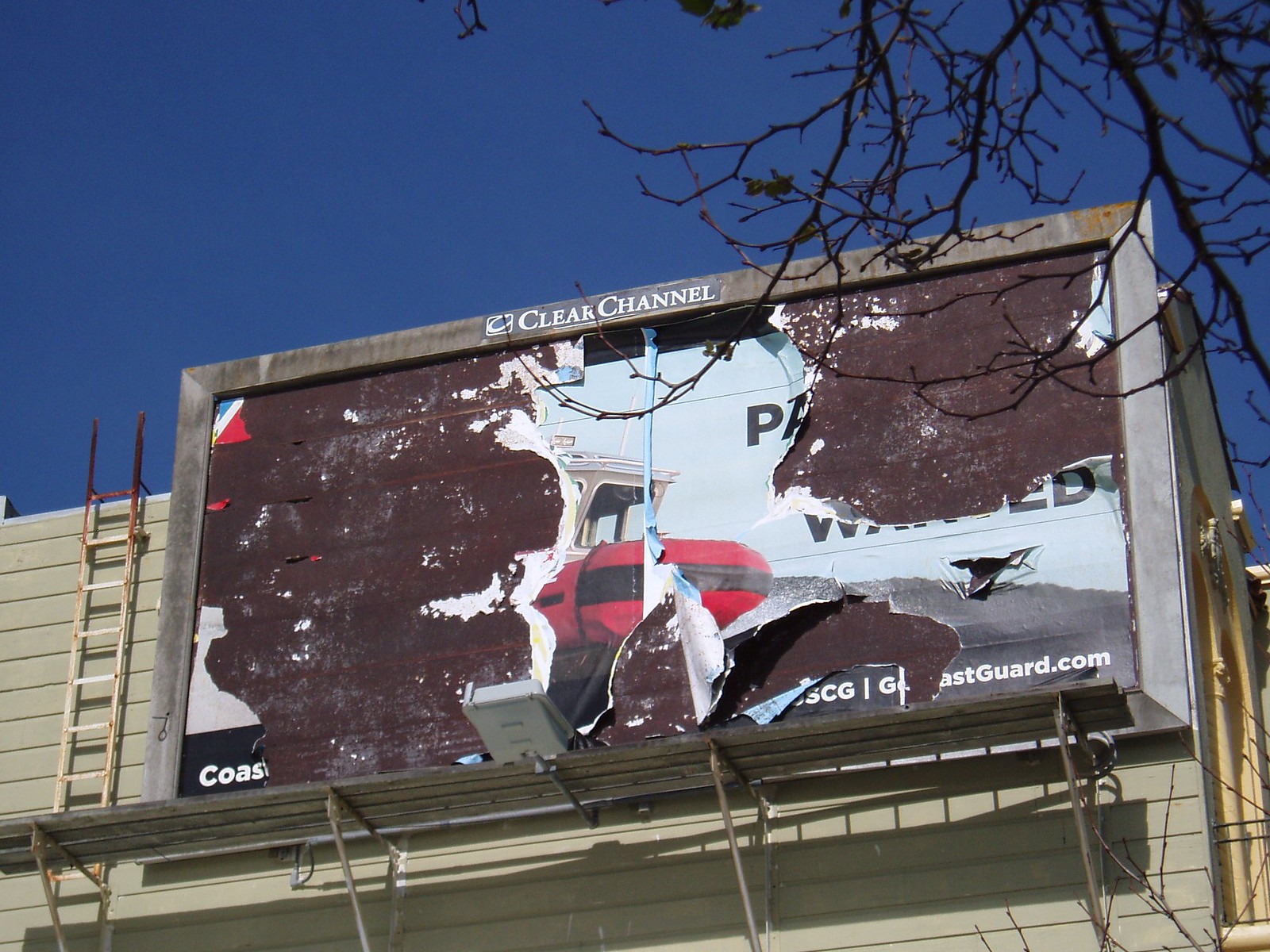This is a detailed color photograph featuring a somewhat close-up view of a weathered billboard mounted on the side of a gray-paneled building. The structure of the building is partially visible, particularly on the left side. Above the billboard, the bright, cloudless blue sky provides a striking contrast to the muted tones of the building. In the upper right corner of the image, a few bare tree branches, devoid of leaves, delicately frame the scene.

The billboard itself shows significant wear, with much of the original image peeled away, leaving only fragments behind. The steel gray frame of the billboard remains intact, and at the top center of the frame, the words "Clear Channel" are prominently displayed in white font. On the lower right corner of the billboard, the website "coastguard.com" is still visibly intact, hinting at the board's original intent. Additionally, a small portion of an image depicting a boat can be discerned, suggesting that the advertisement was once for the Coast Guard.